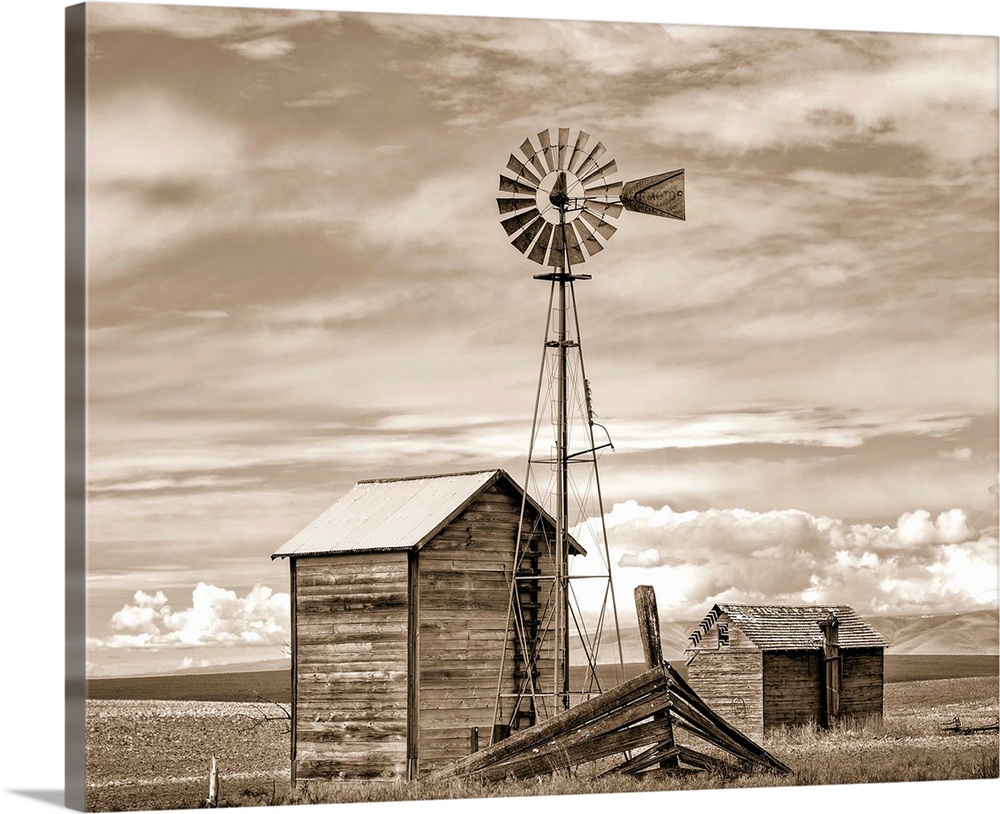This is a detailed black-and-white photograph, possibly of an older vintage, capturing a rustic farm scene. Central to the image is a tall, traditional windmill with a large, circular metal fan and a tail resembling a weather vane. The sky dominates the upper portion of the picture with a mix of billowy white, light gray, and darker clouds. To the left side of the image, partly visible, is the edge of what appears to be a canvas, hinting that the photograph might be a reproduction of a painted scene.

Beneath the windmill, there are two small wooden structures. The one on the left is a narrow, rectangular building featuring horizontally-laid wooden panels and a sloping, A-frame tin roof. Directly behind it, another wooden building is visible, distinguished by its wooden roof and a small chimney protruding from it. Both structures are situated within a barren, flat farming field devoid of vegetation except for patches of brown grass in the foreground.

In the immediate foreground, there's a broken wooden fence with posts and slats scattered about. The horizon shows a row of gentle, rolling hills that enhance the pastoral ambiance. The combination of elements — the structures, the windmill, the sparse vegetation, and the sky — encapsulates a simple yet profound depiction of rural life from a bygone era.